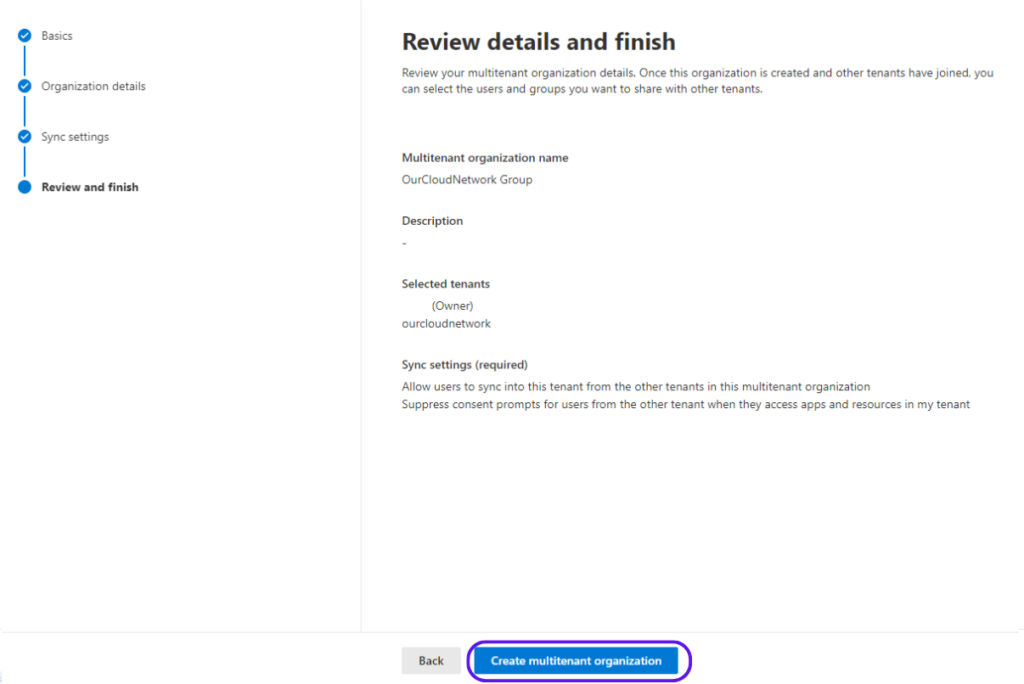The image depicts a user interface with a white background, showcasing a multi-step process for setting up a multi-tenant organization. On the left side, there are five distinct steps labeled "Basics," "Organization Details," "Sync Settings," "Review," and "Finish." Each step is represented by a small blue circle containing a checkmark, connected by a line to illustrate progress. The final step, "Review and Finish," is highlighted with a solid blue circle, indicating the current step.

On the right side, the interface displays in-depth instructions and fields for "Review Details and Finish." The top section instructs the user to review multi-tenant organization details, emphasizing that once the organization is created and other tenants have joined, the user can select specific users and groups to share with those tenants.

Below this, there are several input fields and options:
1. **Multi-Tenant Organization Name:** (Field where the name can be entered)
2. **Cloud Network Group Description:** (Currently blank)
3. **Selected Tenants:**
   - **Owner:** Cloud Network
   - **Sync Settings:** (Required checkbox) 
     - "Allow users to sync into this tenant from the other tenants in this multi-tenant organization."
     - "Suppress content prompts for users from other tenants when they access apps and resources in my tenant."

At the bottom of the interface, there are two buttons:
- A "Back" button to return to previous steps.
- A prominently outlined blue button labeled "Create Multi-Tenant Organization," which initiates the final creation process.